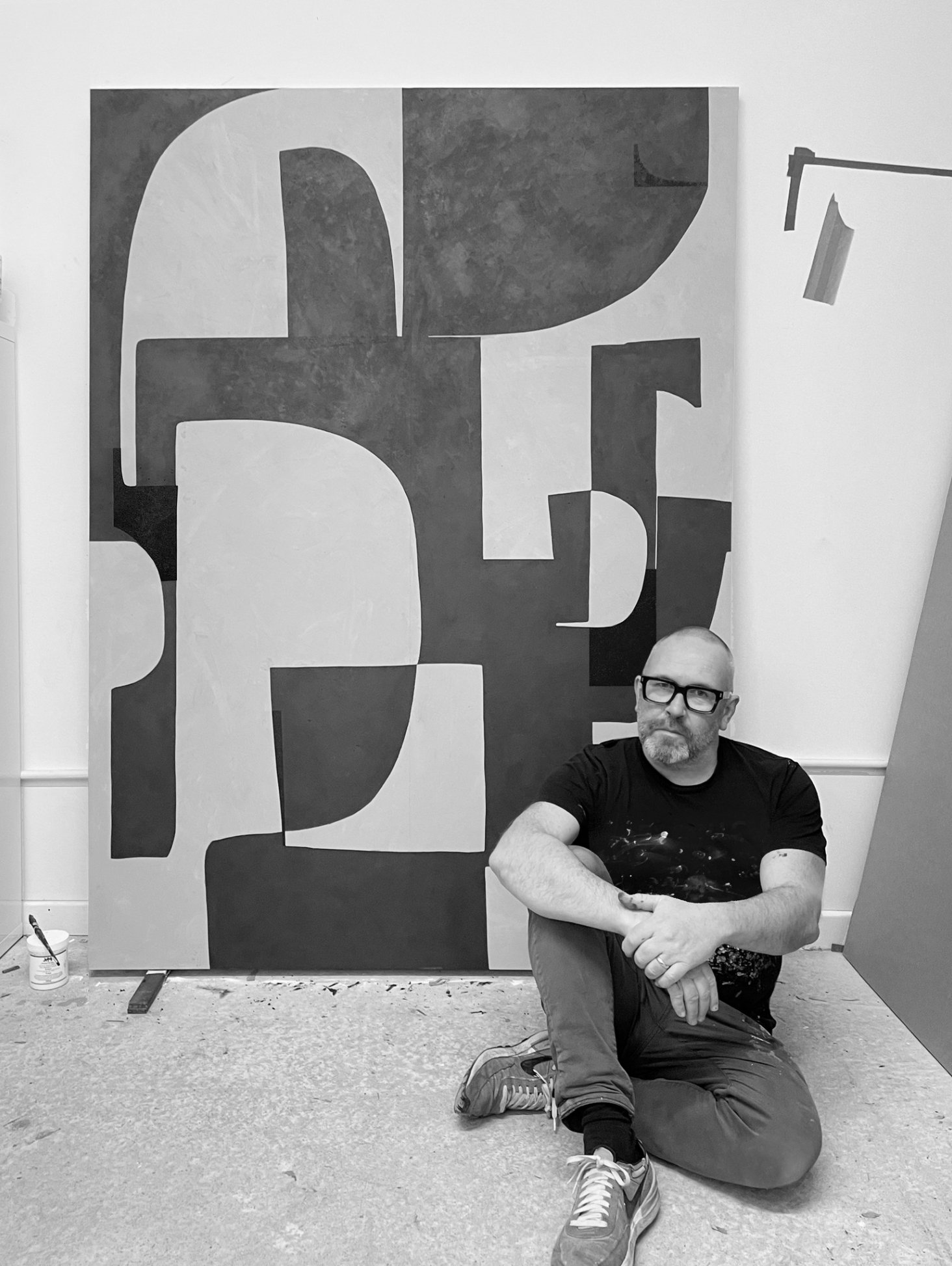This black and white photograph captures a late 40s to early 50s Caucasian man sitting on the floor, positioned in front of a large painting that he appears to be the artist of. The man is bald by choice, has a salt-and-pepper goatee, and is wearing thick-rimmed, dark glasses. Dressed casually, he sports a black t-shirt with indistinct graphics, jeans, black socks, and Nike tennis shoes with white laces. A wedding ring is visible on his finger, indicating he's married.

The setting appears to be a slightly dirty, concrete floor speckled with paint spots. The man sits in a relaxed posture with one knee up, resting his arm on it, and his other leg folded beneath him, almost like a pretzel style. Notably, a paint brush and a paint can are situated in the lower left corner of the image, opposite where he sits.

Dominating the background is his artwork, which measures approximately six feet tall and four to five feet wide. The piece resembles a collage with a black and white geometric design that includes shapes resembling block letters or abstract forms inverted in color. The overall composition suggests an intimate portrayal of the artist in his creative space.